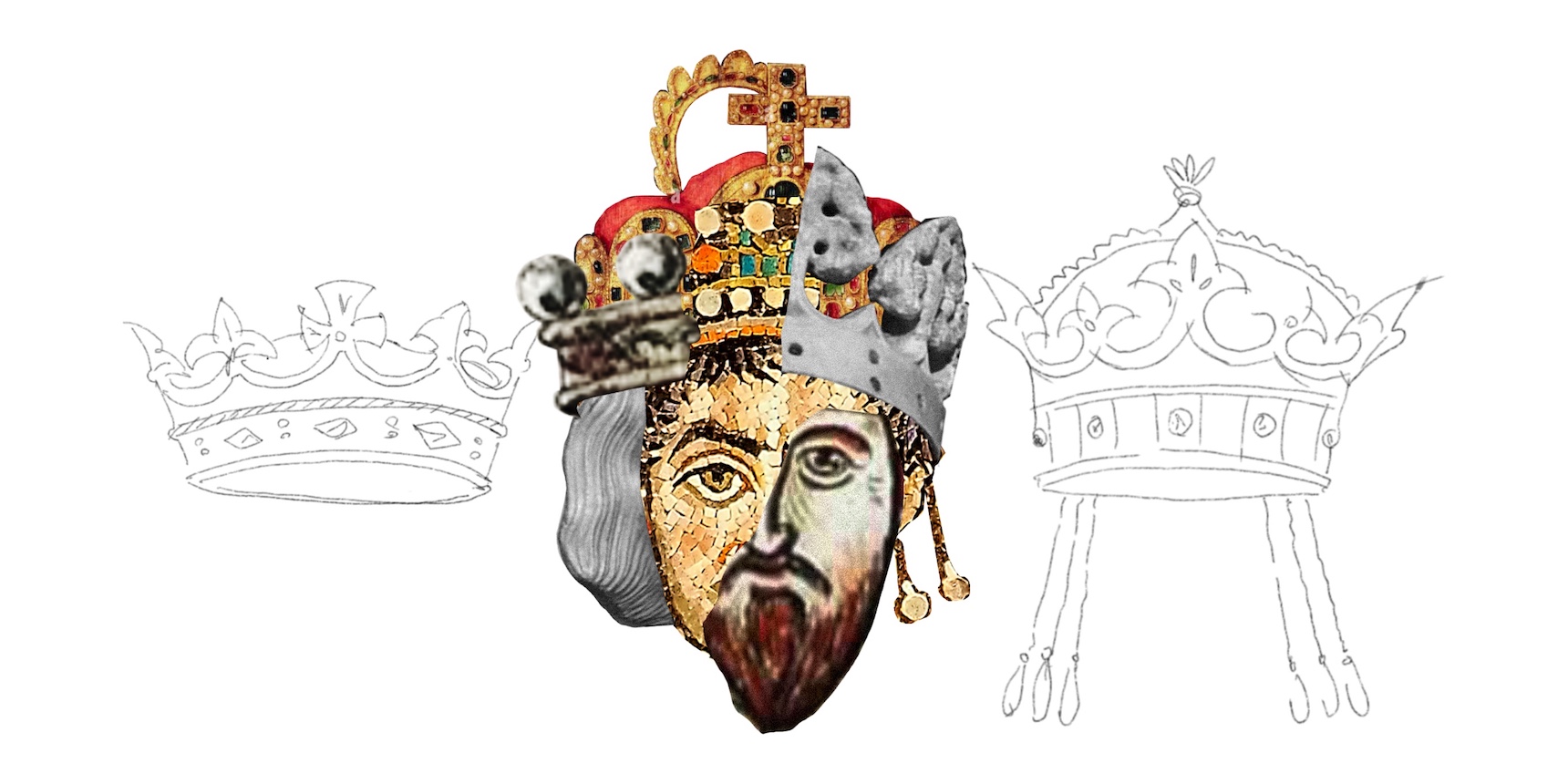This image depicts a striking, highly detailed drawing of a man's face that appears to merge multiple artistic styles into one cohesive representation. The face is split into two distinct halves: the left side is colored in a tan hue while the right side remains white. The man sports a reddish-brown beard and mustache, extending across both sides of his face. Additionally, his eyes and eyebrows differ between the two halves, emphasizing the asymmetrical nature of the design.

Atop his head rests a grand, jeweled crown featuring a prominent cross adorned with several jewels at its center. This crown is partially colored, adding to the intricate detail. To the left of the man's face is a smaller, outlined crown, simpler in design. On the right side, there is a significantly larger and more ornate crown featuring three decorative elements that dangle on either side, drawn in black pen or ink. The entire composition appears as a graphic design or computer-generated image, yet retains a hand-drawn essence, generating a visually compelling and complex portrait.